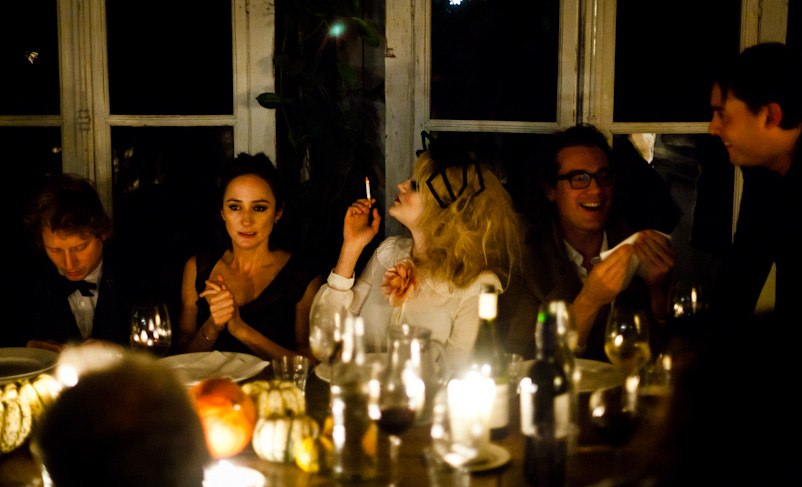This detailed color photograph captures a vibrant evening party inside a dimly lit restaurant, with darkness visible through the wall of windows in the background. At the center of the image is a woman dressed in a white long-sleeved outfit adorned with a prominent orange flower at the neck. She is holding a cigarette in her right hand, and her profile is illuminated as she looks off to the left. To her left, another woman, wearing a sleeveless black ballgown and with her dark hair elegantly styled, sits with hands clasped together. A man in a tuxedo and black bow tie, positioned to the far left, sits with his head bowed.

Further to the right, a gentleman with glasses and clad in a jacket and collared shirt holds a napkin and smiles warmly. Adjacent to him, another man stands at the end of the table, looking down and sharing in the laughter. The table itself is adorned with lit candles, numerous wine glasses, bottles, and dishes, contributing to the ambiance. An obscured head appears in the foreground, adding a layer of depth to the scene.

This photograph, taken in landscape orientation, captures a moment of conviviality and refined elegance, emphasizing the interaction and subtle details of the guests' attire and expressions, bathed in the soft glow of candlelight.